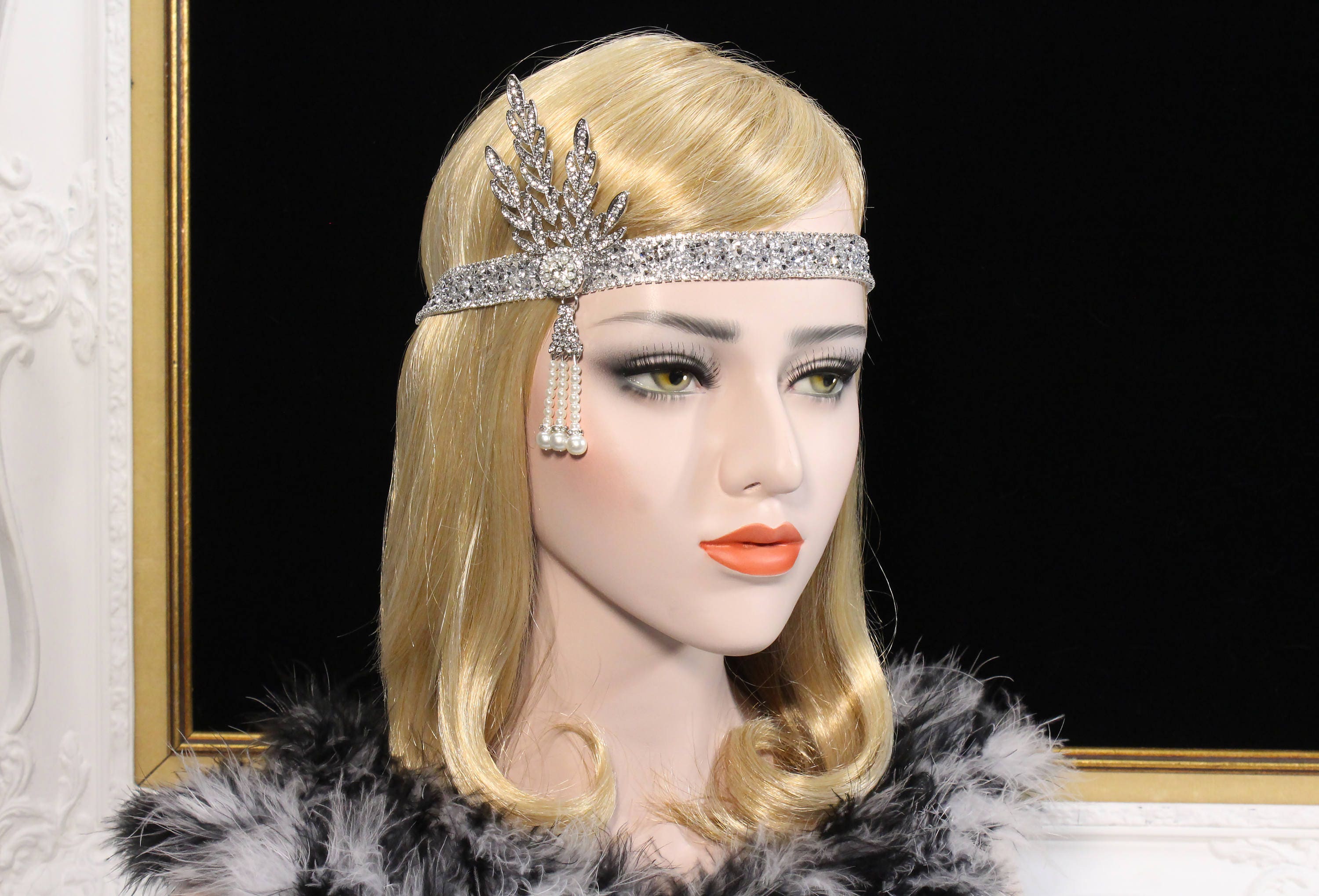The image showcases a close-up of a detailed mannequin or a doll, modeled after a woman. Her head is turned toward the bottom left side of the frame. The scene captures her from just below the shoulders upward, providing a focused view of her attire and features. She is adorned in a striking black and white feathered top, adding a touch of elegance to her appearance. Her blonde hair cascades to her shoulders, beautifully curling at the ends. Enhancing her sophisticated look, she wears a headband with a diamond-shaped design. The background features a blackboard framed with an ornate gold border, adding a sophisticated contrast to the image.